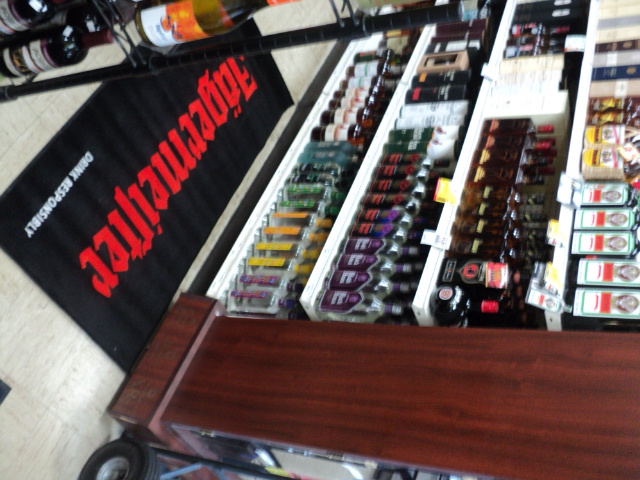The image depicts a small section of a liquor store, oriented sideways. On the floor, there's a black mat with red lettering that reads "Jägermeister," and in white letters below that, it says "drink responsibly." The gray-tiled floor sets the base for the scene. A prominent brown wooden laminated column extends upward beside the mat. Shelves in the background hold a variety of alcoholic beverages: at the very top, there are bottles of Jägermeister. Below these are rows of other brown and clear bottles, followed by bottles with a mix of vibrant labels including purple, red, yellow stripes, and a distinctive black bottle with a red cap. This shelf section is accompanied by another black wire rack with wine bottles labeled in orange, red, and white. To the right, there appears to be a dolly, hinting at restocking activity. The overall setting seems compact but well-stocked, with the entire scene giving a slightly fuzzy and out-of-focus appearance.